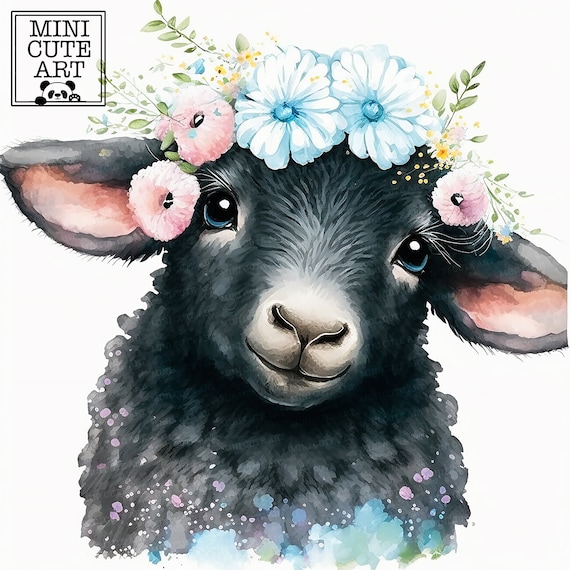The image features a digitally created lamb with a white background. At the top left corner, there is a cube with the text "Mini Cute Art" in black, accompanied by a small, black-and-white panda peeking out from the bottom. The lamb itself is predominantly grey with a white nose and a mouth that is a blend of grey and white. Its ears are pink on the inside and grey on the outside, while its eyes are blue with black pupils and a small white glimmer. The lamb is adorned with a mix of pink and blue flowers in its hair, complete with green leaves and bits of yellow in the flowers. The wool at the bottom of the lamb's neck transitions from blue to pink and finally to grey. The overall composition is visually appealing, combining elements of both illustration and painting, and showcases delicate details such as the white eyelashes of the lamb and the intricate design of the flowers.